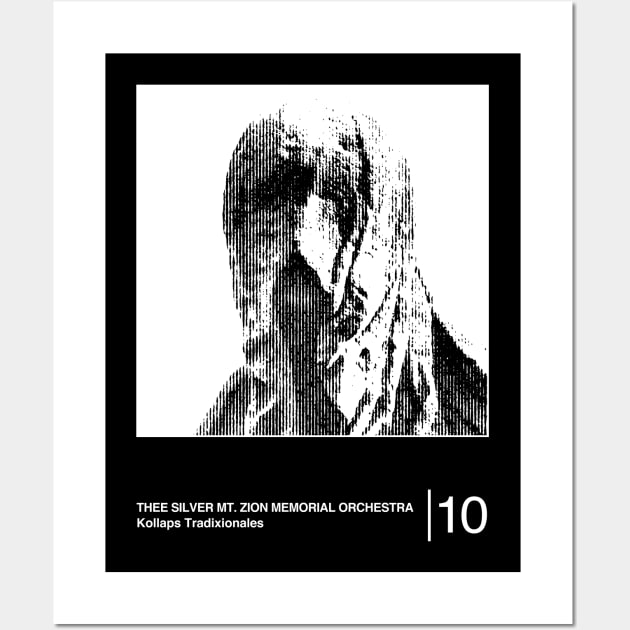The image has a distinct appearance of an album cover or promotional material for the Silver Mount Zion Memorial Orchestra. The design features a centrally positioned black and white photograph surrounded by a black border with a white frame, all set against a light gray background. The photograph itself is somewhat abstract and pixelated, depicting a person shrouded in a white veil or scarf, with shadows and rough shapes distorting their facial features, particularly around the eyes and mouth. This gives the image an eerie or unsettling feel. Below the photograph, in white typeset over a black background, the text reads "The Silver Mount Zion Memorial Orchestra Collapsed Tradicionales," followed by a vertical line and then the number "10." The overall effect suggests a digital rendition or low-resolution artwork, accentuated by vertical lines and areas of white space, creating a haunting visual experience.